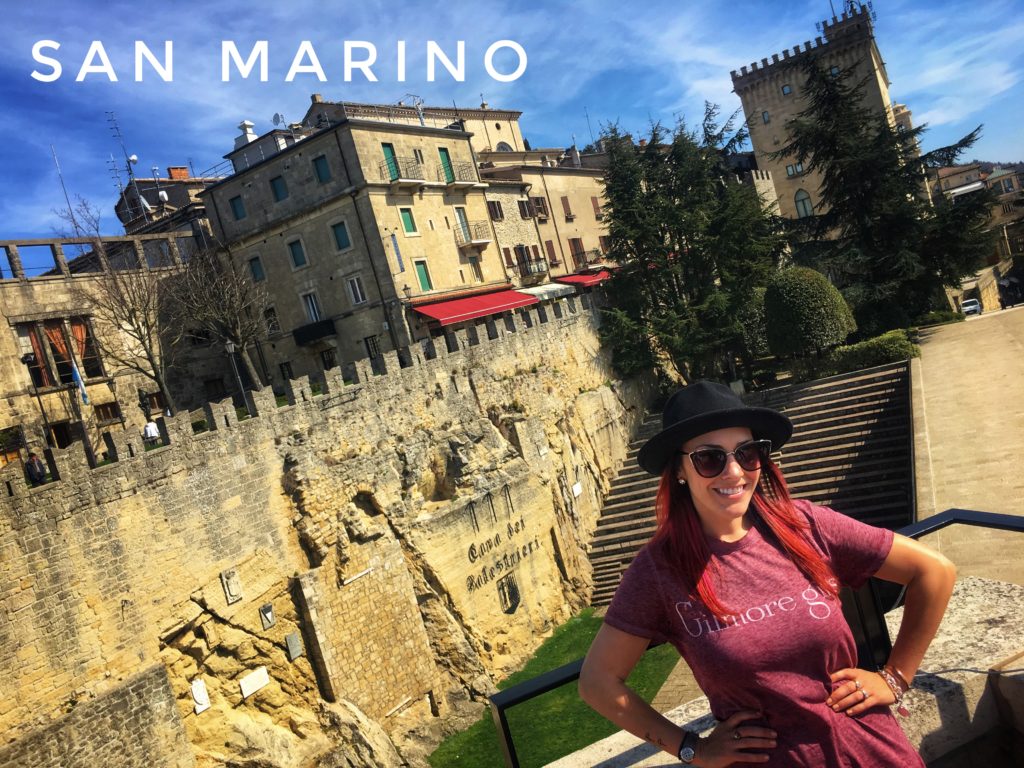In this vibrant tourist photograph, a woman with dyed red hair stands confidently in an urban setting of San Marino, as indicated by the text in the top left corner. Sporting a stylish black hat with a medium brim and wide sunglasses, she exudes a blend of modern flair and casual cool. Her maroon shirt with "Gilmore Girls" emblazoned across the chest adds a pop of color against the backdrop of an old, partially decrepit stone wall adorned with text. The stone wall, featuring a castle-like parapet, separates her from several old multi-story buildings, one of which is notable for its green blinds and red and white striped awnings. The woman strikes a pose with her hands on her hips, revealing a silver earring in her right ear, a watch on her right wrist, and a silver and black bracelet alongside three rings on her left. Behind her, stone stairs ascend the wall, leading up to sculptured bushes and evergreen trees, partially obscuring a castle tower structure in the upper right corner.